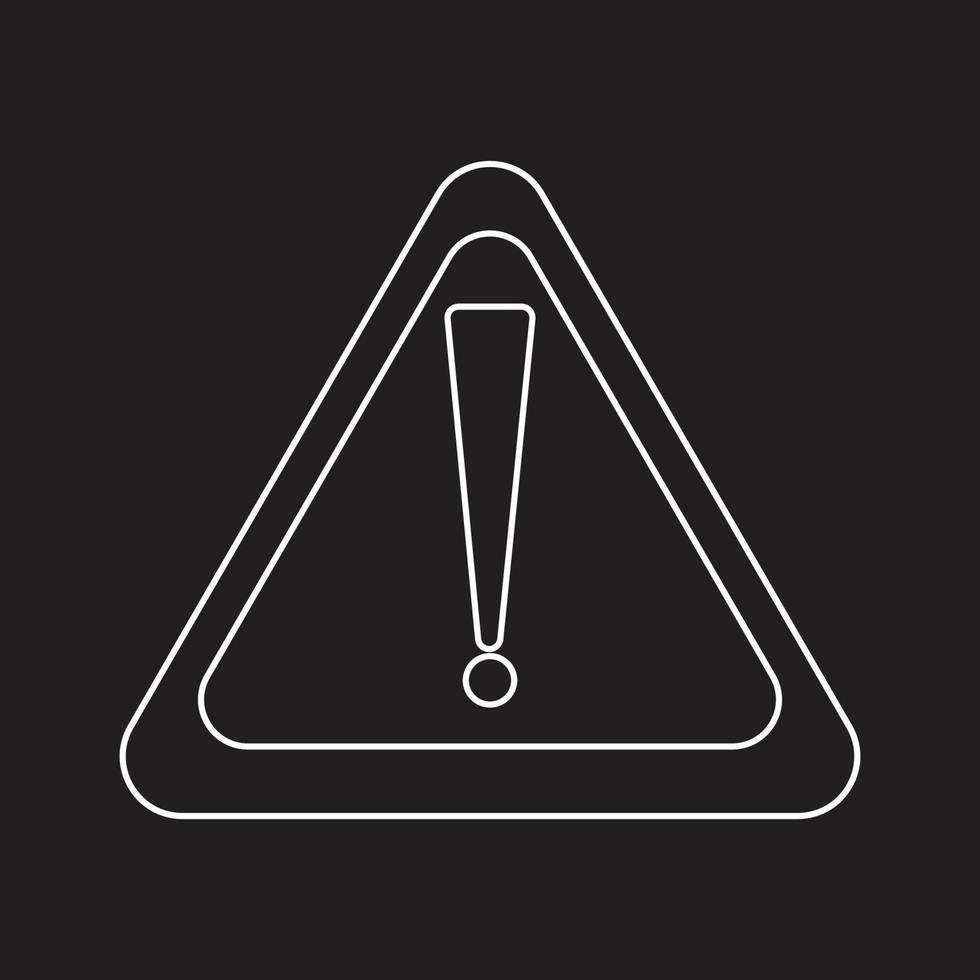The image features a stark black background with a central symbol drawn in white lines. The symbol consists of a larger triangle with slightly rounded corners, outlined in a thin white line, enclosing a smaller triangle also outlined in white. These triangles are nested within each other, both filled with black in between. Inside the inner triangle, there's a prominent exclamation point, also outlined in a thin white line. The overall design forms a distinct contrast with the black background, creating a simple yet striking visual of nested triangles and an exclamation mark, centrally positioned within a black square frame.